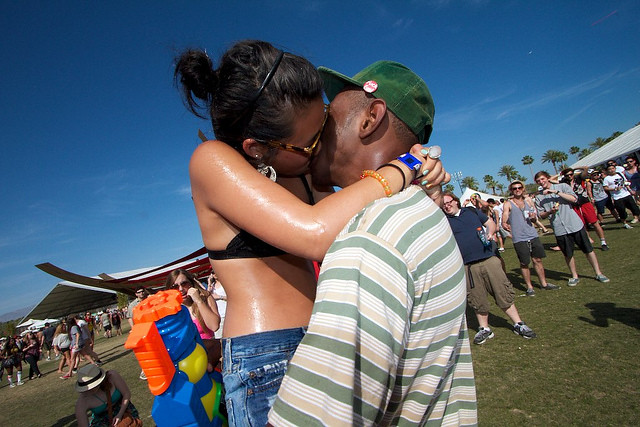At an outdoor concert festival, possibly Coachella, a striking image captures an intimate moment between two central figures who seem to be African American. In the vibrant, sun-soaked scene filled with the blues of the sky and greens of the grass, the couple stands out: the woman, dressed in a black bikini top and denim bottoms, has her hair up and shields her eyes with sunglasses, passionately kissing a man to her right. The man, possibly Tyler, the Creator, is distinctive with his green hat adorned with a button, and a gray, white, and tan striped shirt. Around them, festival-goers are captivated, some taking pictures, others smiling and pointing, adding to the festive ambiance under a clear blue sky dotted with resilient tents.